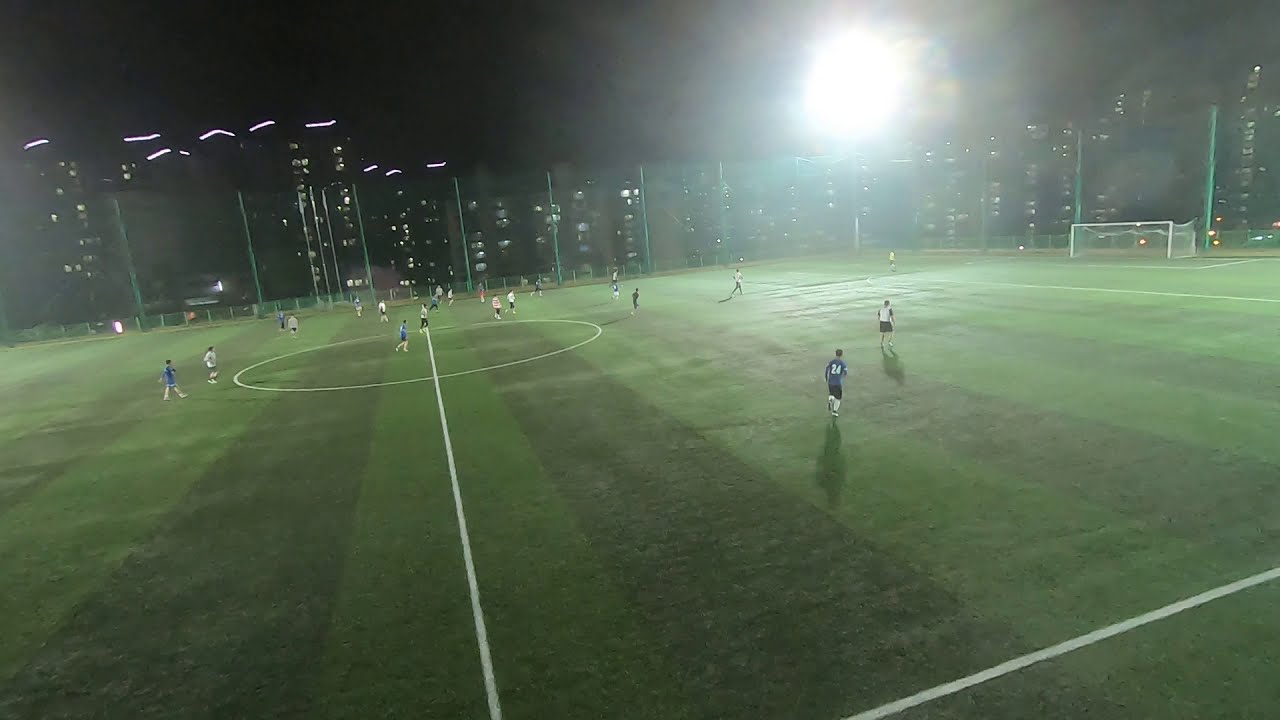The photograph captures a night-time soccer match on what appears to be a massive, professional stadium with a soccer field accentuated by alternating stripes of light and dark green turf. The field is surrounded by towering fences designed to keep the ball in play. Near the upper right of the image, a blindingly bright area light casts a sun-like glare, obscuring parts of the scene with a light flare. The teams are easily distinguished by their uniforms, with one team in blue jerseys and the other in white. The players look tiny due to the distant camera angle, emphasizing the vastness of the field. On the left side, big stadium lights illuminate the entire scene, and behind the fence, a backdrop of apartment buildings looms. One goal is barely visible in the upper right corner, and the goalie stands far from it. The field features a large center circle, but the other goal on the opposite end is not visible due to the perspective. Scattered figures mill around, though they are too far away to discern their actions clearly.